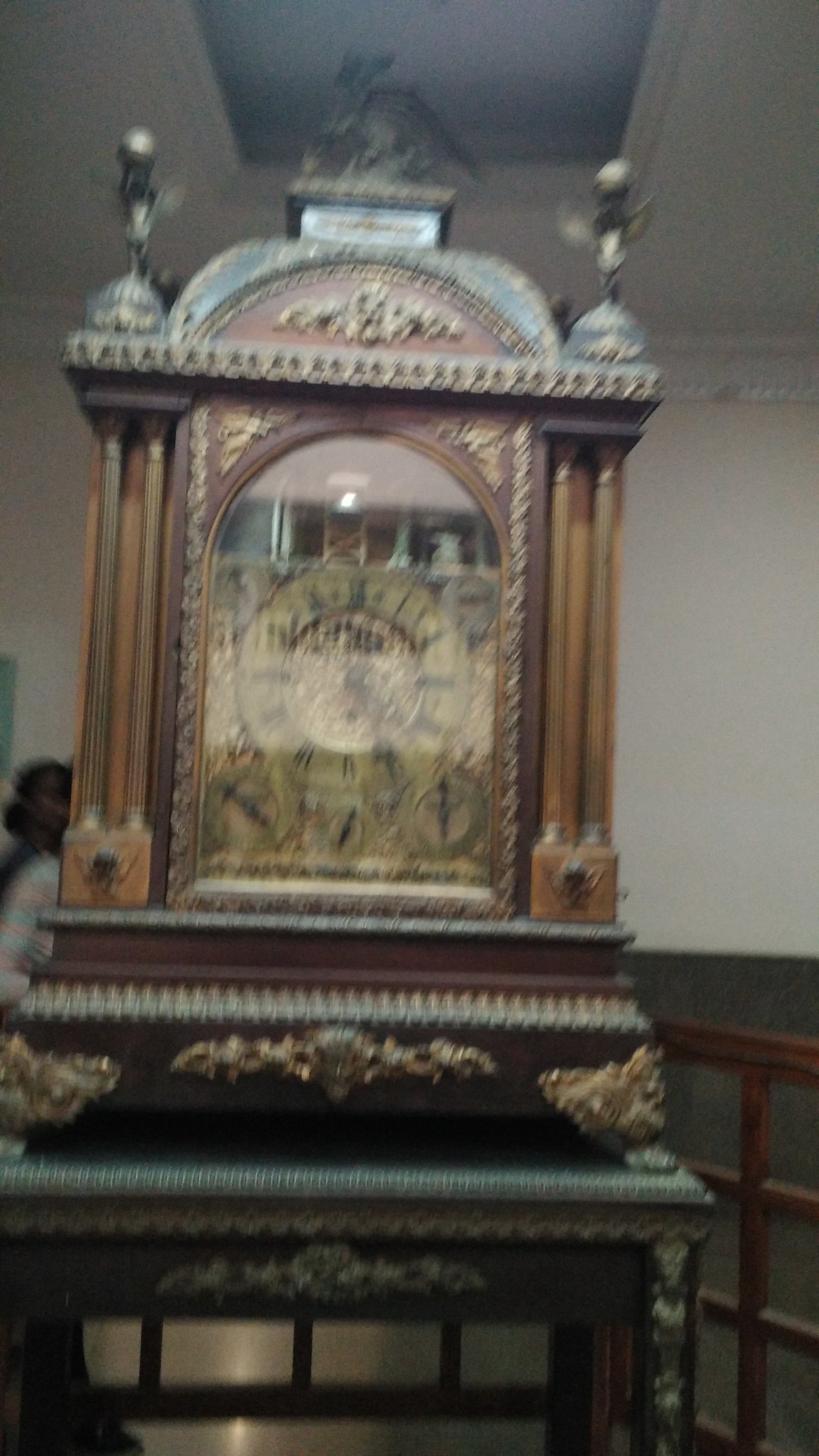This photograph, though slightly blurry, captures a striking antique-style clock located inside a building that resembles a museum with its tall, high ceilings. The clock, an exquisite artifact, showcases a fusion of Asian and old English design elements, possibly even Indian. Made primarily of dark wood, it features intricate metal accents in bronze or gold tones that add to its ornate appearance, though the blur makes it difficult to discern the finer details.

On either side of the clock are two metal columns that frame its structure. The clock’s face, crafted from metal and protected by a glass window, adds a traditional touch to its overall aesthetic. Topping the clock are several statues or ornaments made of metal, adding a grand and decorative finish to this historical timepiece. Despite the image's lack of sharpness, the grandeur and detailed craftsmanship of the clock are unmistakably evident.